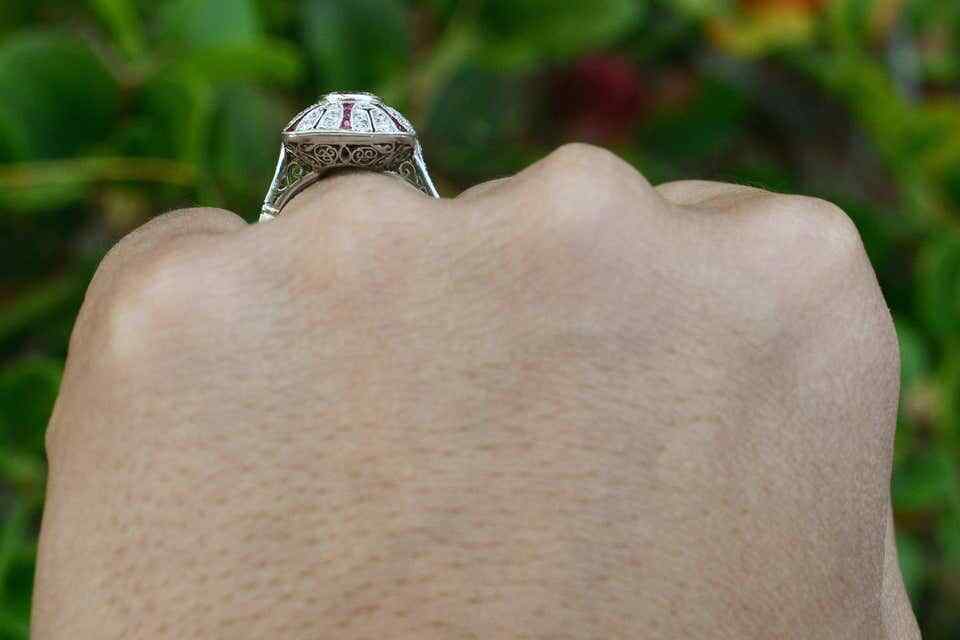This close-up image centers on a Caucasian man's left hand, showcasing the back of his fist with noticeable detail. The hand appears recently shaved, revealing visible pores and prominent knuckles accentuated by the positioning of the thumb, confirming it is the left hand. The fingers are curled into a fist, with a silver and white ring adorned with faint scarlet accents on the ring finger. The design of the ring, visible from the side, suggests it might be a class ring, though its full form is not entirely discernible. The background features a blur of tropical plants and flowers, placing the sharply focused hand in stark contrast against the vibrant yet obscure backdrop, making the hand the clear focal point of the image.